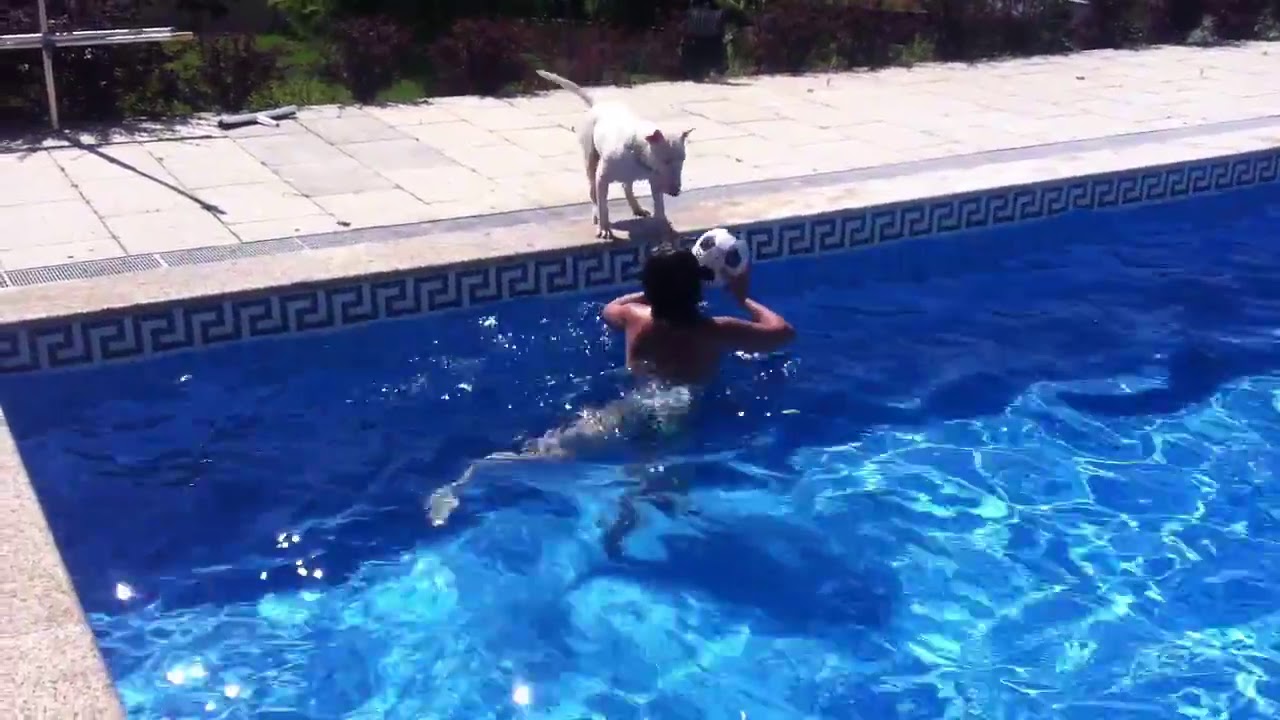The image captures an outdoor scene in the middle of the day, featuring a person in a sizable swimming pool positioned towards the bottom of the frame. The person, who appears to be a topless man with black hair and facing away from the camera, is holding a soccer ball. Their upper body is above the water. At the edge of the pool, a white dog with short hair and a straight, medium-length tail is standing on a deck or patio, attentively looking down at the man and the ball. The deck consists of square white stones arranged in a grid pattern, bordered by rougher stone. Beyond the deck at the top of the image, there are some bushes and patches of grass, adding a touch of greenery. The overall scene portrays a relaxed, bright outdoor setting with prominent colors including different shades of blue, white, tan, black, gray, green, and purple.